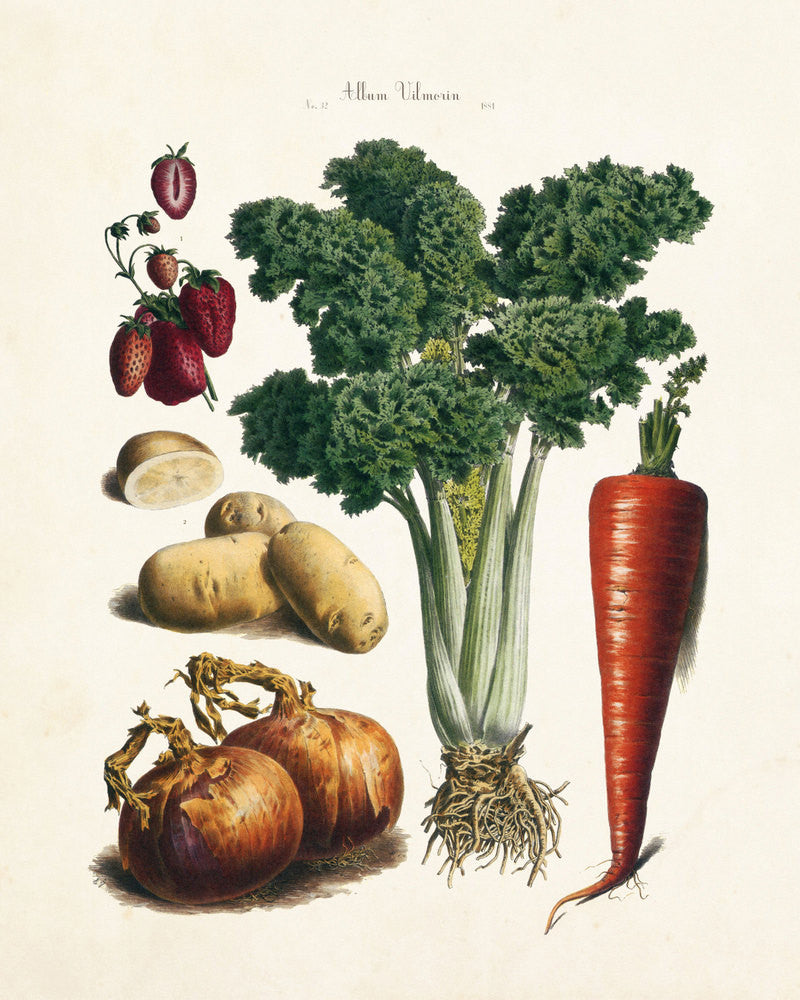This artwork, set against a calming beige background, showcases a vibrant assortment of garden vegetables. The top of the piece is adorned with the inscription "Albem Ville Marin." Central to the illustration is a meticulously detailed stalk of celery, its green leaves extending upwards while the roots dangle below. To the right beneath the celery lies a strikingly orange carrot, its leafy green top left intact, radiating freshness. In the lower left corner, two onions are depicted with their outer peel layers and tops still on. Positioned to the left of the celery are three sturdy baking potatoes. Completing the ensemble, the upper left corner features an elegant plant stem bursting with ripe, red strawberries, adding a touch of vivid color to the earthy composition.